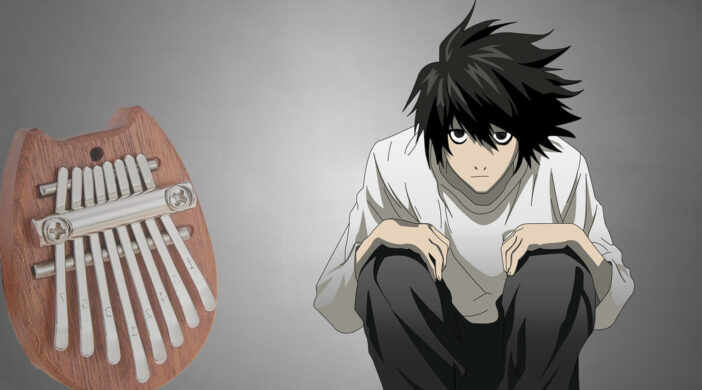This is a large rectangular anime-style poster set against a gradient background of gray and white. Dominating the right side of the poster is a serious-looking anime character named L from the series Death Note. L is depicted kneeling with his hands placed over his knees, looking directly out of the image with large, intense black eyes set in a triangular, pointy-chinned face. His black hair is spiky and parted to the right, and he is dressed in a white long-sleeve shirt and black pants, portraying a slightly disheveled appearance.

To the left of L is a small, simplistic musical instrument, identified as a kalimba. It features a wooden base with a distinctive shape resembling cat ears at the top. The kalimba has eight silver keys attached to a bar at the top, secured by two large screws. Beneath these keys, a metal bar is visible, and a hole is drilled in the middle of the wooden surface. This layout suggests that the poster might serve as a visual reference or a tutorial thumbnail for playing a specific theme song from the Death Note series on the kalimba. The detailed contrasts and elements of both the character and the instrument create a unique and intriguing composition.